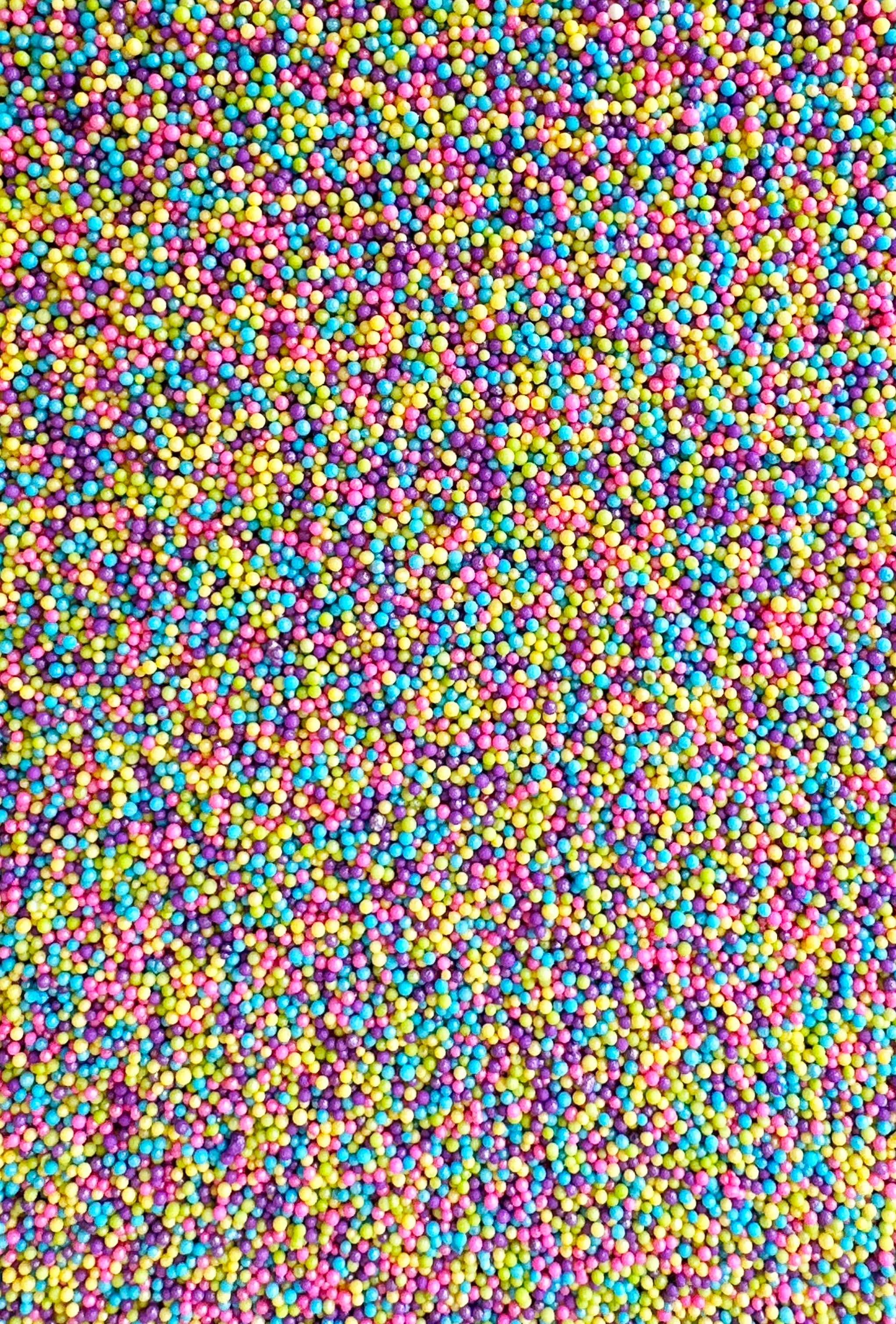We have a detailed image depicting a densely packed sea of very small, vibrant beads in assorted colors including purple, yellow, pink, blue, and teal. The beads, which cover the entire image without any background or text, are distributed haphazardly, creating an abstract, mosaic-like pattern. With its bright and well-illuminated quality, the photograph exudes a sense of organized chaos and vivid artistry. Despite their appearance resembling candy such as Nerds, it is more likely that the image was generated using AI, lending it a hyper-realistic yet surreal aesthetic. The scene could evoke comparisons to up-close views of sprinkled confections or intricately beaded jewelry, highlighting its richly detailed and colorful composition.